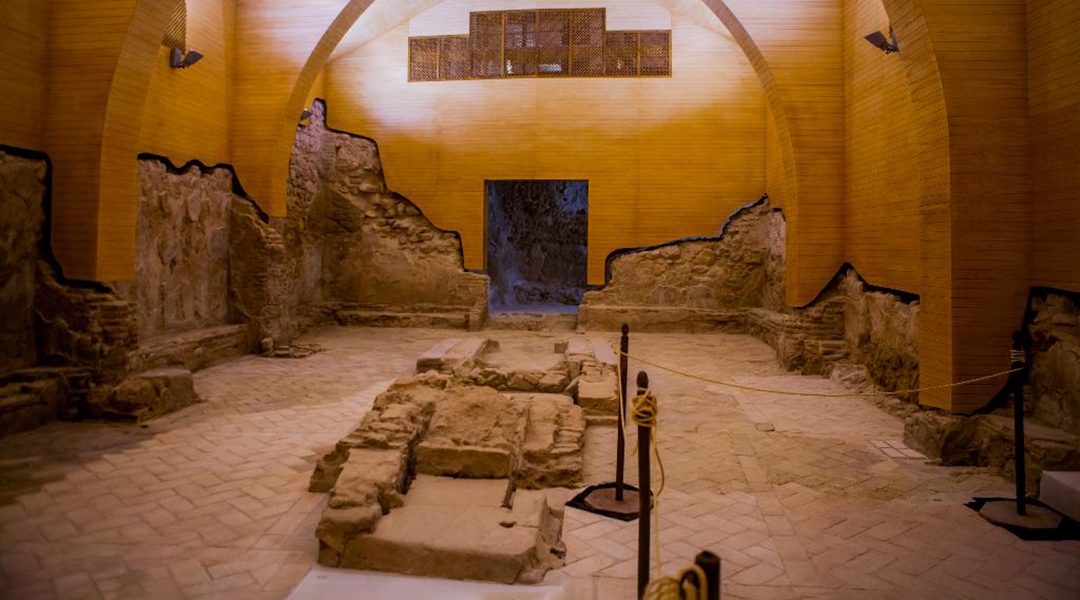The image depicts the interior of an ancient ruin, possibly Egyptian or from a similar era of antiquity. The cavernous room features elaborate architectural details, including arches and columns, distinguishing it from a typical basement. The lower portion of the walls is comprised of exposed beige-colored stone and brick, while the upper section transitions into a wooden veneer, possibly mimicking bamboo slats, giving it a golden sheen. The light brown stone floor is scattered with large slab stones and is roped off with yellow chains attached to black poles, indicating it's an area for observation. The center of the room houses a platform or pile of brown stones. In the background, there is an archway leading to a dimly lit, rocky area, adding to the ambiance of an ancient temple.